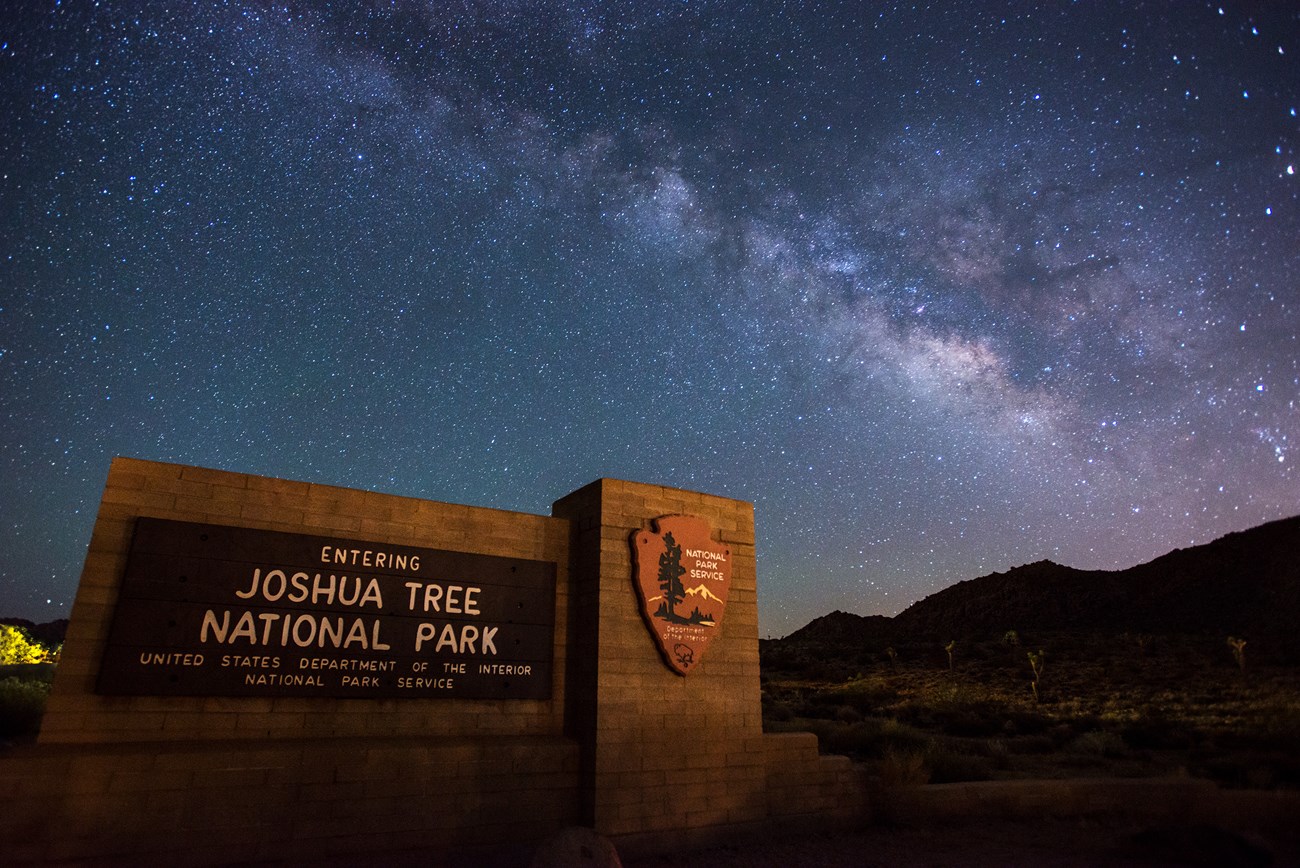This evocative nighttime photograph captures the breathtaking beauty of Joshua Tree National Park under a resplendent starry sky. Dominating the foreground is a prominently lit sign mounted on a substantial brick structure that warmly declares, "Entering Joshua Tree National Park, United States Department of the Interior, National Park Service." To the right of the text, the iconic arrowhead logo of the National Park Service is proudly displayed, adorned with a picturesque depiction of a pine tree, majestic mountains, and a noble bison. The sign stands as a guardian at the park's entrance, nestled in the semi-darkness that envelops the surroundings.

The sky, covering the majority of the image, is an astral masterpiece, likely captured with high dynamic range to showcase an astounding expanse filled with countless stars and the mesmerizing Milky Way. The background gradients from vibrant blues to deep grays, occasionally punctuated by wisps of nebulous clouds. This celestial panorama bathes the scene in a palette of ethereal colors, enhancing the photograph's dreamy allure.

Complementing the grandeur above, the landscape below unfolds in subtle, shadowy tones. To the right, a silhouetted mountainscape provides a dramatic contrast, while hints of vegetation dot the landscape, partially illuminated by ambient light. The detailed and multi-exposure effect of the photograph keenly captures both the starkly beautiful sign and the infinite cosmos, portraying a tranquil yet awe-inspiring entrance to one of America's cherished natural treasures.